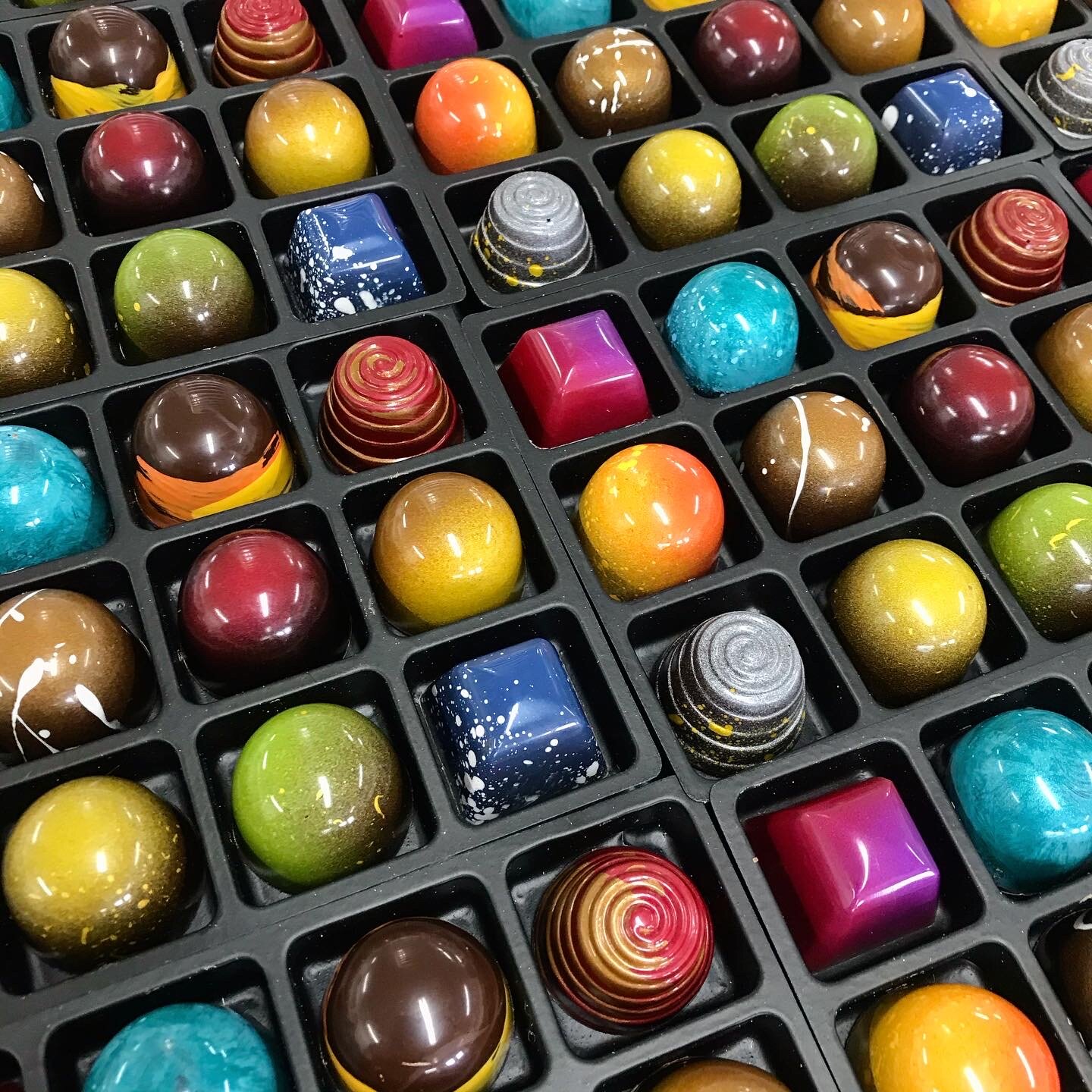The image showcases a close-up of various colorful and ornate objects, resembling either rocks, gems, or intricately designed chocolates. These items are meticulously arranged in a black, sectioned container akin to a box for chocolates, with individual compartments. The vibrant collection includes shades of greenish-blue, teal, purple, navy blue with white spots, red, silver, orange, light green, and beige. Some of the items display swirly patterns, while others are either perfectly round or square in shape. Notably, one object at the bottom left looks like a chocolate donut, featuring a brown top and lighter underside. The entire assortment is housed within black trays, emphasizing the diverse and shiny appearance of these visually striking pieces.